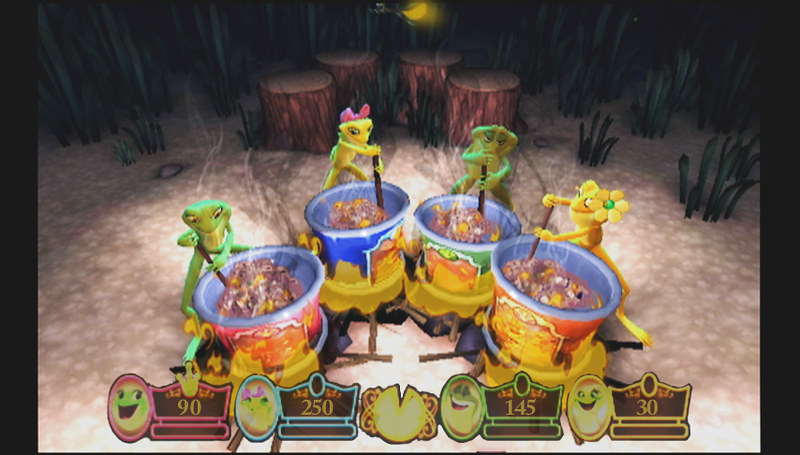The image depicts an in-game screenshot from an early 2000s-era multiplayer video game featuring four characters that resemble colorful, anthropomorphic lizards or geckos. Each character is positioned around a large, vividly colored cauldron—red, blue, green, and orange—placed over campfires. These characters seem to be engaged in a minigame where they earn points by stirring concoctions in their respective cauldrons. The character in blue appears to be leading with 250 points, while the other characters lag behind. Their progress and score are indicated by icons and status bars at the bottom of the screen. The setting is a woodland area with tall grass and tree stumps in the background, adding a rustic nature vibe to the scene. The ground has a white, speckled appearance, reminiscent of snow. Despite the dated graphics, the game exhibits a charming and colorful visual appeal, making it look playful and engaging.